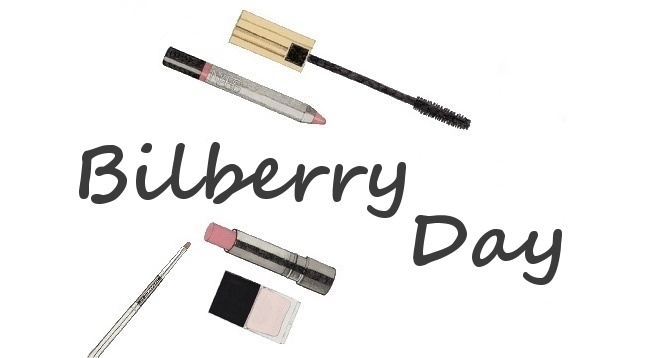The image showcases a variety of makeup tools arranged meticulously against a completely white background. At the top, there is a black mascara brush with a gold lid alongside a makeup pencil, which features a pink end, a silver section, and a black tip. Centered between these items is playful, comic-style grayish text that reads "Bilberry Day." Below the text, the bottom section includes a silver stick brush on the left, a pink lipstick in a silver tube in the middle, and a see-through plastic bottle containing pink powder on the right. The aligned positioning of these six beauty essentials—mascara, pencil, brush, lipstick, and powder encapsulates a well-organized display, punctuated by the whimsical 'Bilberry Day' inscription.